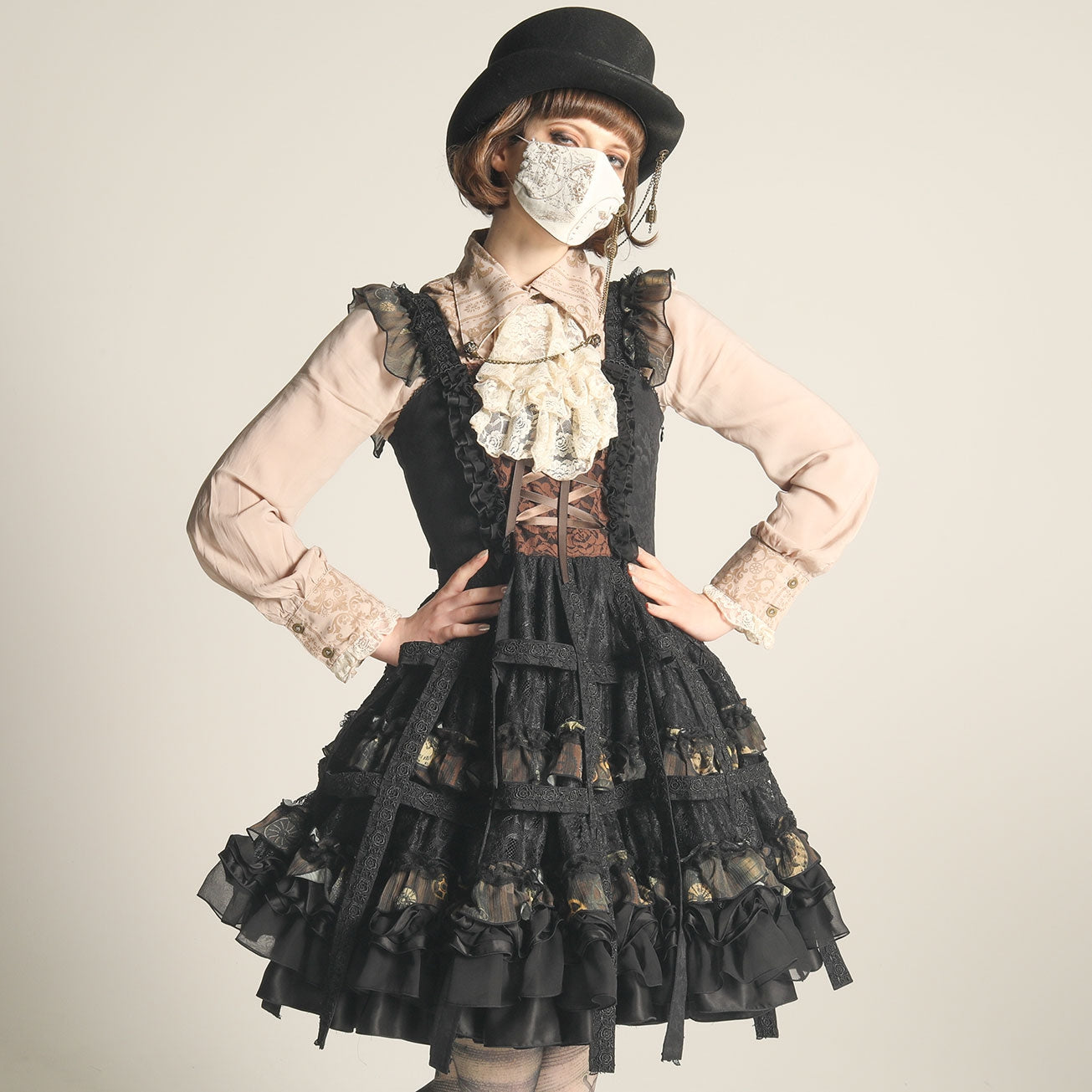This is a posed photograph of a woman in an intricate, steampunk-inspired Victorian outfit, captured against a tan background that darkens towards the bottom. She sports a black top hat above her curly auburn hair, which features brown bangs. Her face is partially covered by a white surgical mask adorned with a floral design, allowing only her eyes and neck to be visible. 

The focal point of her attire is a black dress that marries Victorian frills with cyberpunk elements, extending from her shoulders to just above her knees. The dress includes a black bodice with tan and brown laces, and it features a standout red velvet sash and a white cloth in the front. Her puffy skirt, adorned with blue-black ruffles and intertwined straps, adds volume, finishing just above her knees where the image cuts off. 

Underneath the bodice, she wears a tan blouse with long, pinkish-white sleeves that culminate in doily-type cuffs, each fastened with two brass buttons. Adding a touch of elegance, a white, doily-looking scarf peeks from beneath her collar. The ensemble is completed with visible stockings underneath the skirt, enhancing the vintage yet futuristic aesthetic.